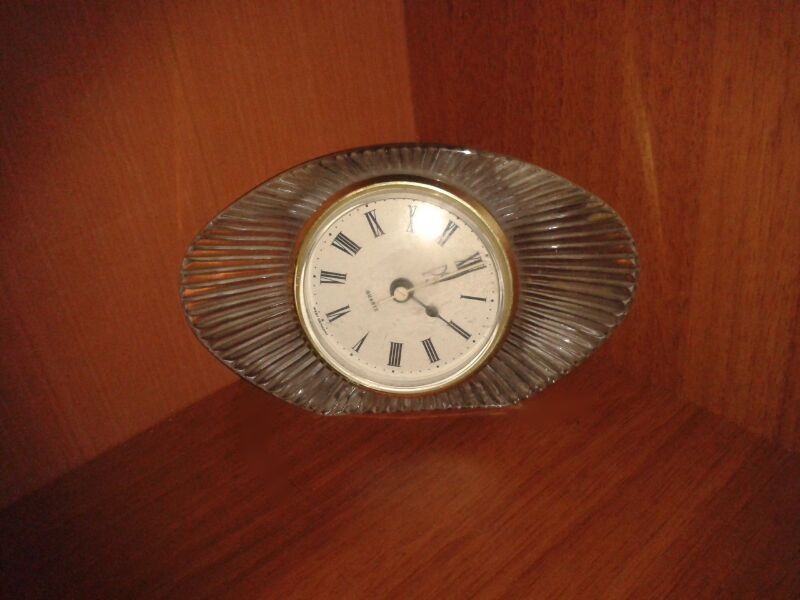The image features a close-up, indoor color photograph of an old-fashioned clock, likely from the 60s or 70s, situated in the corner of a wooden structure. The setting appears to be the inside of a bookcase or a wooden shelf with dark mahogany wood, evident by the visible grain and rich brown color of the wood surrounding the clock on three sides — the back, left, and bottom. The clock itself is mounted within an oval-shaped, glass or crystal frame that has horizontal striations emanating outward. The oval frame's transparency allows glimpses of the background.

The clock's face is round, white with black Roman numerals, and encircled by a gold bezel. The hands are black, but the second hand is white, pointing to 12. There's a discrepancy noted in the angles, with the 12 o'clock position twisted almost to the upper right, indicating the clock might be misaligned in its mount. The time displayed is about 4:11, with the big hand on the 11 and the small hand on the 4. The photo is slightly grainy and out of focus, with some flash glare visible on the upper part of the clock's lens.